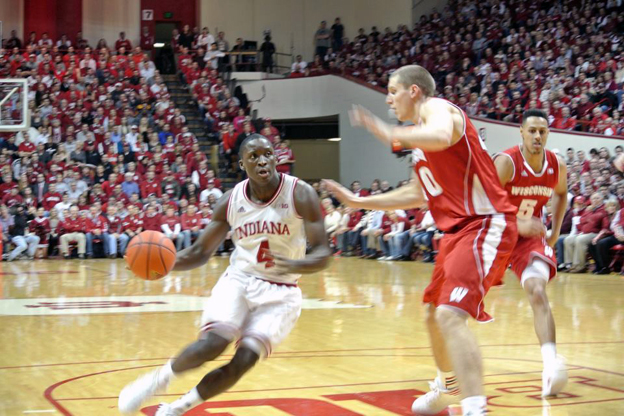The photograph captures an intense moment during a basketball game between Indiana and Wisconsin teams. Centrally framed, the image features three key players in action on a shiny, logo-adorned hardwood court. The player on the left, dressed in a sleeveless white jersey with "Indiana" and the number 4 in red, paired with knee-length white shorts and white shoes with tall socks, is mid-run holding an orange basketball. Opposing him are two Wisconsin players in red sleeveless jerseys with white trim, and the numbers 10 and 5 in white, respectively. Their red shorts also feature white stripes down the sides. One Wisconsin player is actively trying to block the Indiana player. The background reveals rows of spectators filling the bleachers, adding to the high-energy atmosphere of the indoor basketball court. The scene is vividly colored with predominant hues of white, red, orange, tan, and brown, capturing the dynamic and competitive spirit of the game.